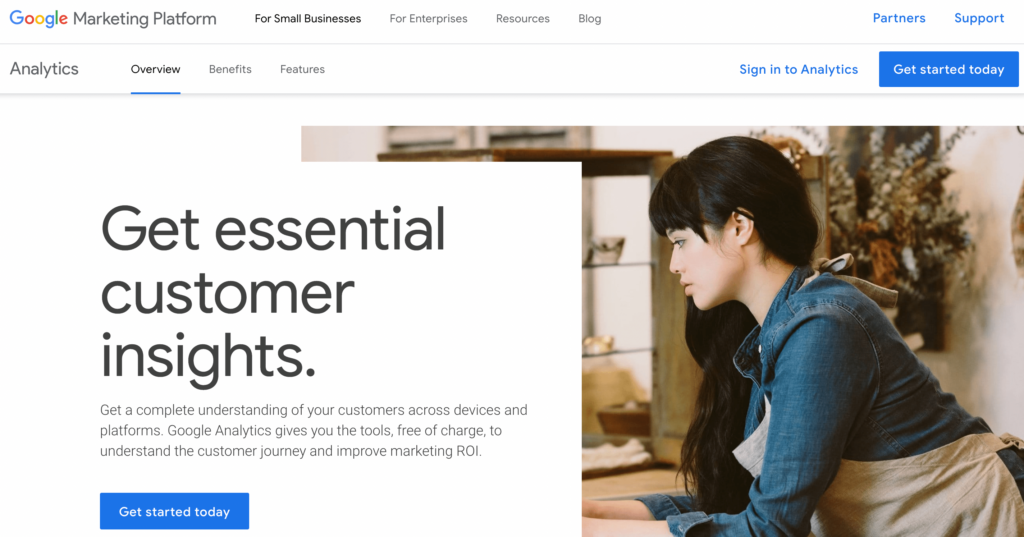The image prominently features the text "Google Marketing Platform," with the word "Google" displayed in its iconic colors—blue, red, yellow, blue, green, and red—while "Marketing Platform" is written in gray. Below this title, there are navigation options for "For Small Businesses," "For Enterprises," "Resources," and "Blog," suggesting these are clickable links in a real-life setting. To the right, in blue text, are additional options labeled "Partners" or "Support," and beneath them, the prompt "Sign In to Analytics" is visible.

A blue banner on the right side of the image features the white text "Get Started Today." Below the banner, headings such as "Analytics," "Overview," "Benefits," and "Features" appear on the left, separated by a fine gray line running horizontally across the image. The "Overview" section is underlined in blue.

In the main content area, the text reads: "Get Essential Customer Insights" in bold black text on a white background. Beneath this, gray text explains, "Get a complete understanding of your customers across devices and platforms. Google Analytics gives you the tools free of charge to understand the customer journey and improve marketing ROI."

Another blue banner at the bottom reiterates "Get Started Today" in white text. 

Adjacent to the text, there's an image of a girl with long, wavy black hair draped over her right shoulder and bangs. She is wearing a long-sleeved, blue button-down shirt with a beige apron. The background suggests she is in a room with beige walls and dried flowers, adding a cozy and professional environment to the scene.